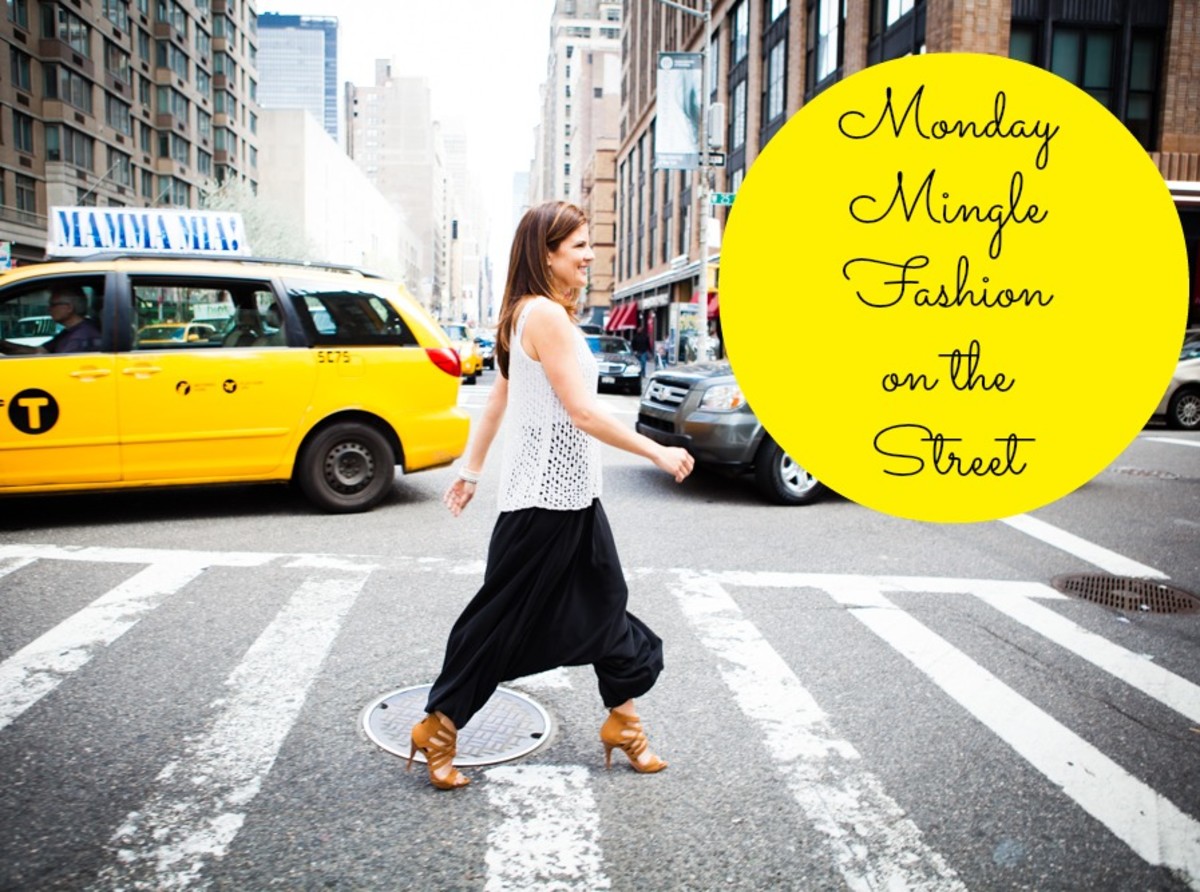This photograph, likely taken in New York City, captures a young woman crossing a busy street. She is walking from left to right within a well-marked white crosswalk, her stride confident and carefree. Wearing light brown strappy high-heeled shoes, a black skirt that reaches her ankles, and a white, lacy sleeveless top, she exudes a blend of elegance and casual chic. Her long brown hair flows gently as she smiles, adding to the vibrant city’s atmosphere. 

At her side, a yellow taxi minivan, showcasing an advertisement for the movie "Mamma Mia!" on its roof, moves through the scene. The juxtaposition of her modern fashion against the classic New York street setting is striking. In the upper right-hand corner of the image, a perfectly round yellow circle stands out, emblazoned with the words "Monday Mingle Fashion on the Street" in bold capital letters. 

The background is a tapestry of New York City elements: various high-rise buildings in shades of brown, white, and light-colored stone, some with numerous windows, others with distinctive architectural details. Behind her, the street pulses with life, cars moving or waiting, a typical scene of urban hustle and bustle. Near her feet, a manhole cover and another grate embedded in the asphalt add a touch of gritty city realism to the composition. This detailed snapshot not only highlights the woman’s fashionable ensemble but also encapsulates the essence of a dynamic New York City day.